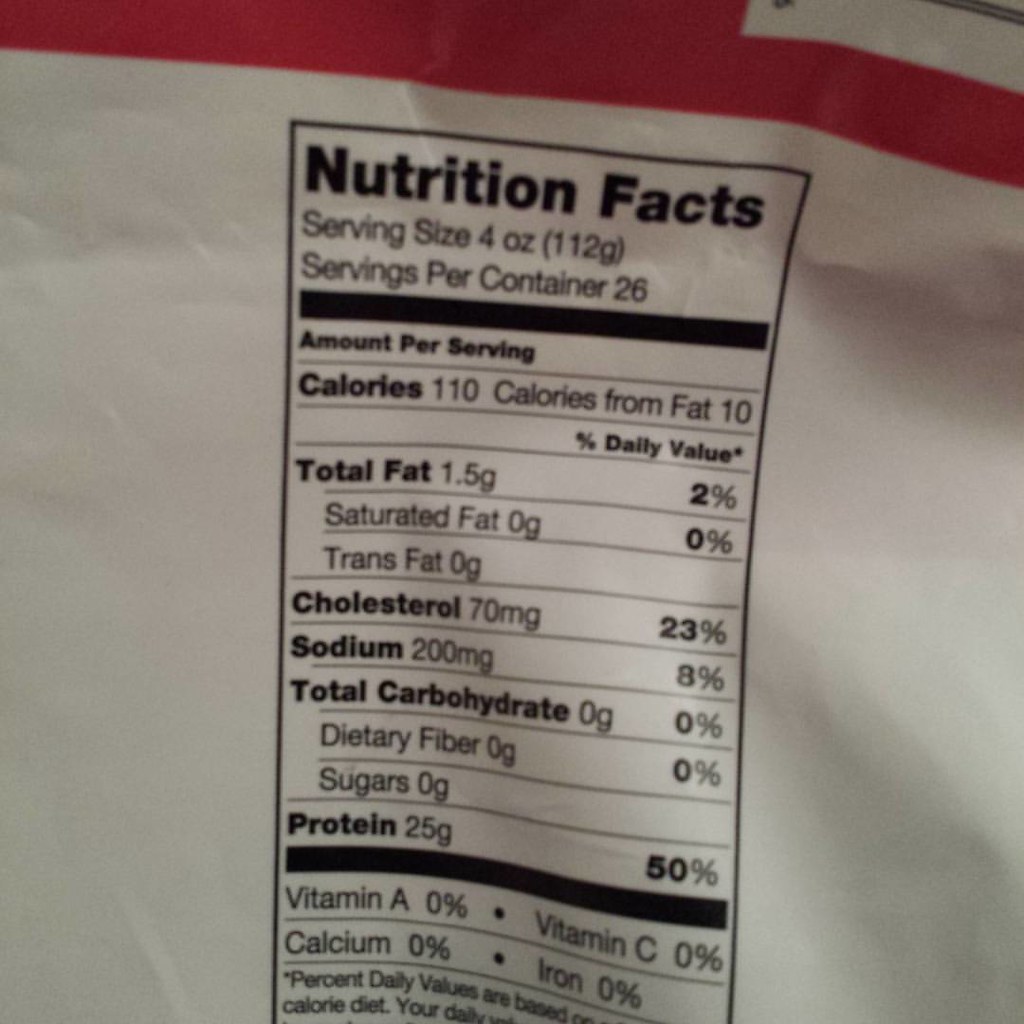The image is a close-up of the nutrition facts label on a food package, which is white with a prominent red stripe at the top. The label lists the serving size as 4 ounces (112 grams) and notes there are 26 servings per container. Each serving contains 110 calories, with 10 calories from fat, totaling 1.5 grams of fat (2% of the daily value). The label does not list any saturated or trans fats. It shows 70 milligrams of cholesterol and 200 milligrams of sodium per serving. There are zero grams of carbohydrates but a substantial 25 grams of protein (50% of the daily value). Additionally, the label indicates that the product contains 0% of vitamin A, vitamin C, calcium, and iron. The footnote on daily values is included at the bottom of the label. Though the specific food item is not identified, it is clear that the package is designed to hold a significant quantity of the product.